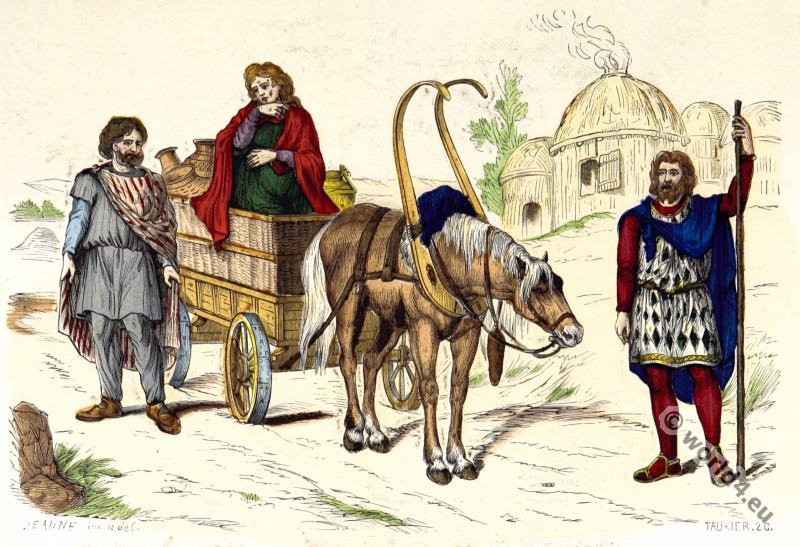The image is an illustration or painting depicting a medieval scene featuring four vividly colored characters contrasted against a muted background. On the far right stands a man in ornate clothing—a blue cape over a white tunic decorated with green diamonds, paired with red pants and holding a long shepherd's stick. To his left, a beige horse with a white mane and tail pulls a wagon. The woman in the wagon, surrounded by pots, wears a green dress and is draped in a red cape. Standing next to the wagon is another man dressed in a gray tunic and pants, with a white cape adorned with red stripes. In the background, several houses with smoke rising from their roofs can be seen, all set against a dirt trail.